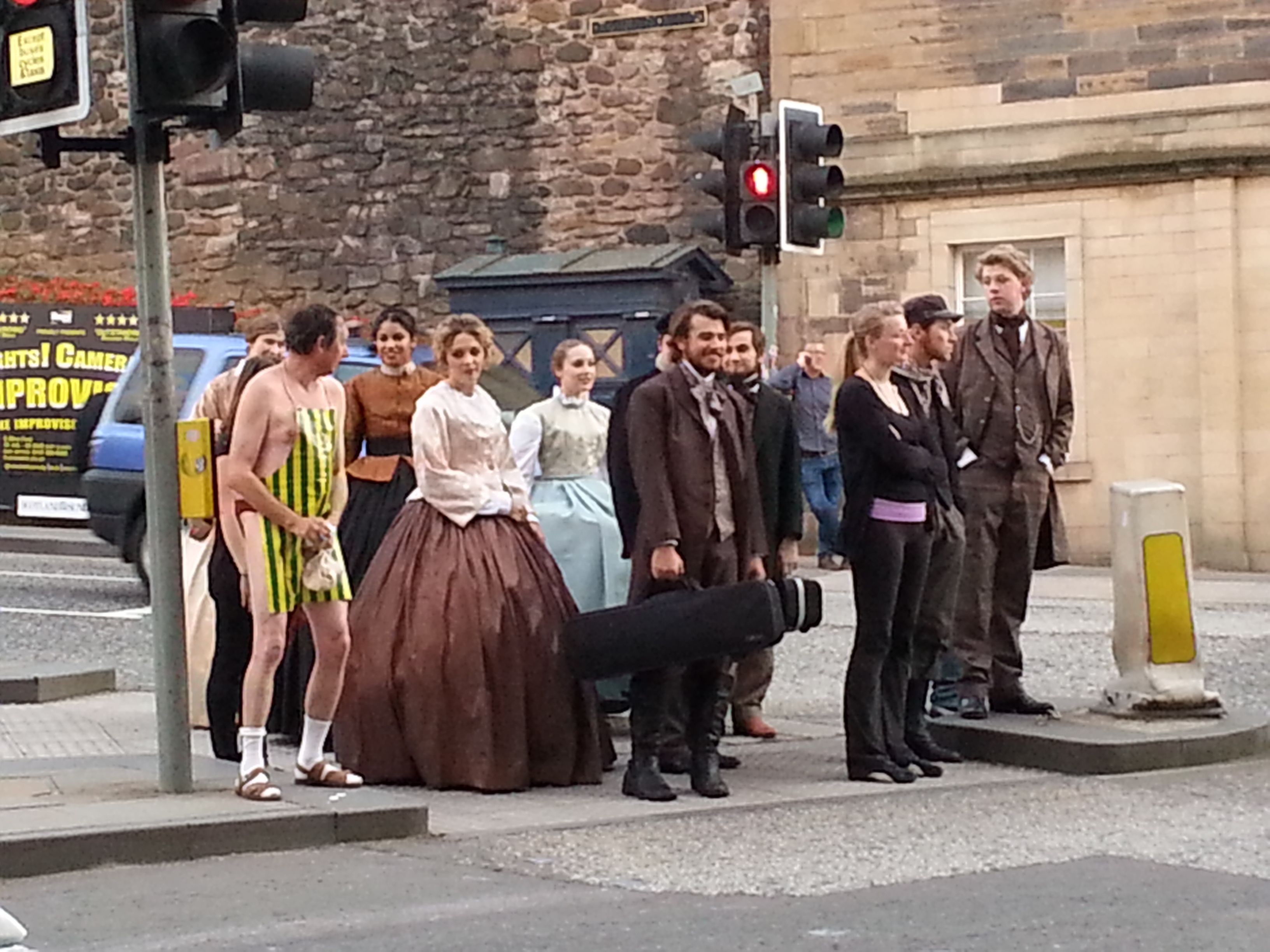The image depicts a scene where a group of people, many dressed in old-fashioned costumes reminiscent of the 1800s, are gathered on the street, seemingly about to cross. On the left, there is a stone wall with brownish and lighter tan sections, and beside it, there is a tan wall with gray and tan blocks above it and a window below. The people are in front of this building, presumably at the back of the picture, and appear to be involved in some form of theatrical or comedic performance. Among them, one man stands out, wearing only a small apron over what appears to be underwear or possibly a speedo, paired with white socks and slippers. Other individuals in the group hold musical instruments, while women are dressed in elaborate, puffy dresses. The scene includes a modern blue car parked in a nearby parking lot, adding to the juxtaposition of the historical attire and contemporary elements.